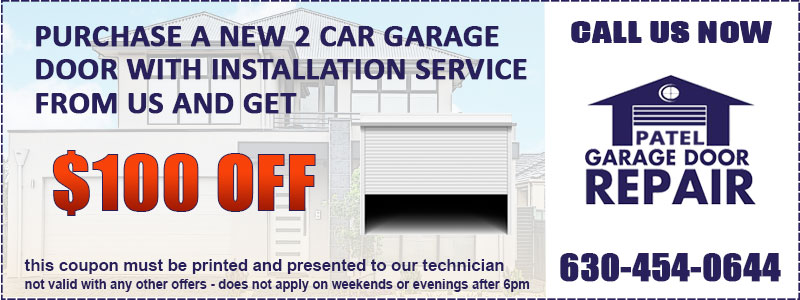This display advertisement, likely sourced from a website, spans a rectangular shape approximately two and a half times wider than it is tall. 

On the left side, a prominent headline in blue, all-caps font reads: "PURCHASE A NEW TWO-CAR GARAGE DOOR WITH INSTALLATION SERVICE FROM US AND GET." Below this headline, in very large red font, it declares: "$100 OFF." 

The background is a very light illustration of a typical two-story suburban home, featuring the garage door in a delicate shade of gray. 

On the right side, the background transitions to white, where text in the same blue, all-caps font commands: "CALL US NOW." Directly below this, the company name "PATEL GARAGE DOOR REPAIR" is displayed alongside their logo—a clean and simple drawing of a garage door with a house. 

At the very bottom of the ad, the company’s contact number is provided: "630-454-0644."